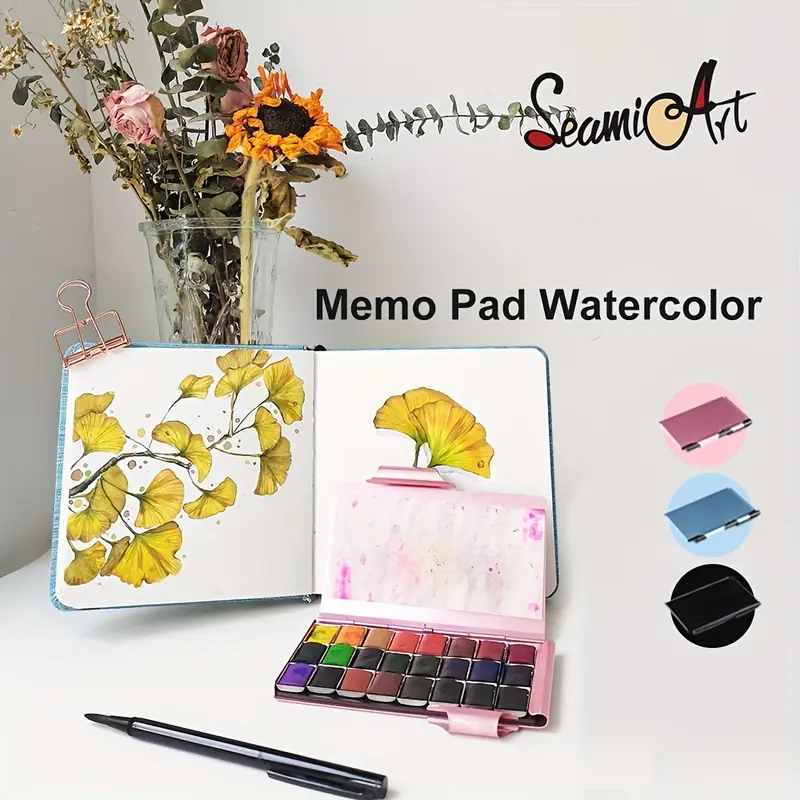The image is an advertisement for a watercolor memo pad, presented on a two-toned background that transitions from tan to white in the lower left. Central to the composition is an open blue-covered journal featuring a captivating watercolor painting of a plant with fan-shaped yellow and green leaves, showcasing exceptional artistry. The journal is held open with a light pink metal clip and is accompanied by an open watercolor set displaying a spectrum of vibrant colors, ranging from yellow to purple and various shades of brown. Positioned in front of the watercolor set is an open black pen, resembling a Sharpie. In the background, a vase filled with dried flowers adds a natural element to the scene.

On the right side of the image, there are three closed examples of the memo pad in pink, blue, and black, each with a corresponding pen. The text "See Me Art" and "Memo Pad Watercolor" appears to float above the vase and on the right side, likely added digitally. The overall setup creatively emphasizes the practical and artistic appeal of the watercolor memo pad.